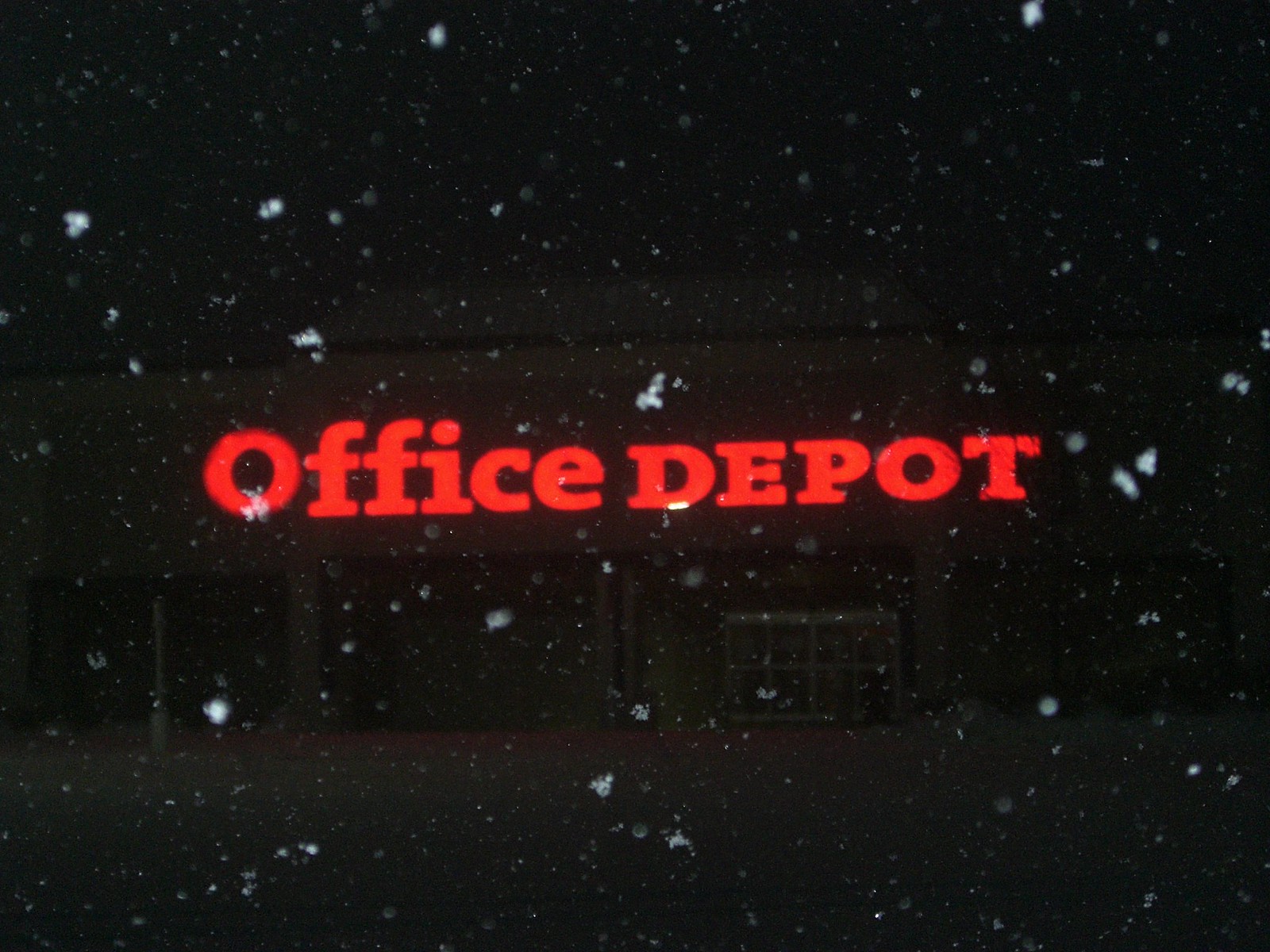The image depicts the exterior of a building set against a dark gray to black gradient sky, which is adorned with a pattern of white dots resembling falling snowflakes of various sizes and brightness levels. The foreground features a structure with eight windows, each framed in white, supported by gray pillars. The bottom section of the image is a solid blackish-gray color, providing a stark contrast to the illuminated building facade. A sign reading "Office Depot" in prominent orange text is prominently displayed on the building. Above the structure, the night sky extends seamlessly into a deep black.